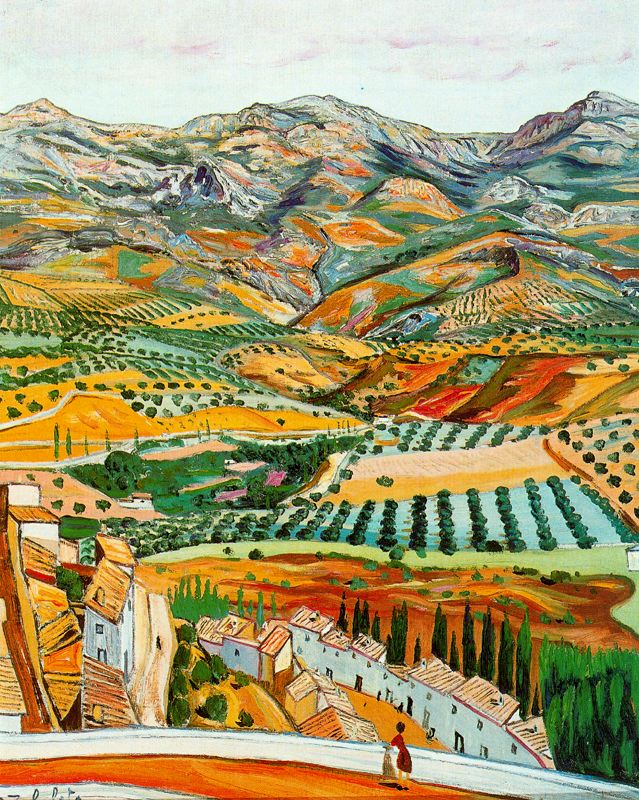This vibrant Van Gogh painting captures a sprawling, colorful landscape with a clear blue sky and purple-tinged clouds over a range of mountains that stretch across the horizon. In the midground, the land transitions from flat, cultivated fields with orderly crops to rolling hills adorned with lush greenery, bushes, and trees, punctuated by bursts of yellow and green, characteristic of Van Gogh's style. The foreground is dominated by a village of white houses with brown or tan roofs nestled amid the foliage. A lone girl in a red dress stands next to a small white wall at the closest point in the image, gazing out over the scenic vista, possibly photographing it. The painting's vibrant palette, featuring greens, oranges, reds, yellows, and blues, creates a lively scene imbued with Van Gogh's distinctive, expressive touch. The artist’s signature is discreetly placed in the bottom left corner.